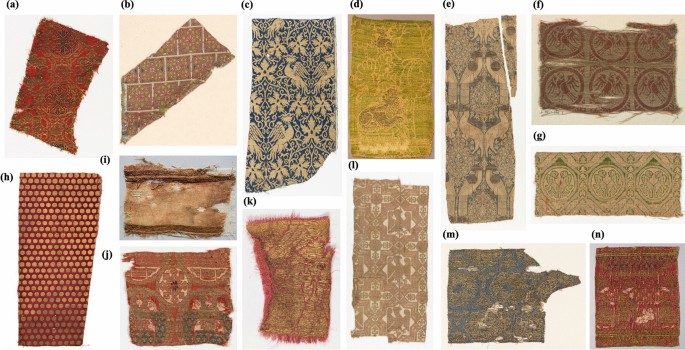This image features a detailed color photograph of various cloth samples, each distinctly tattered and labeled from A to N. These remnants appear weathered, suggesting they are quite old. The fabric pieces are arranged in a grid-like format, with each sample showcasing unique designs and colors.

- **A**: A small rectangular piece of red fabric adorned with a goldish pattern.
- **B**: A fabric with a brownish brick print pattern.
- **C**: A blue and white strip featuring birds and flowers.
- **D**: A golden-green and tan strip with elaborate illustrations.
- **E**: A tan-colored fabric with an intricate design.
- **F**: Gray fabric with circular designs and intricate patterns.
- **G**: A fabric with three circles, each topped with a knob.
- **H**: Red fabric featuring pale-colored dots in a hexagonal pattern.
- **I**: Significantly tattered brown piece with a darker border.
- **J**: Another red piece with tapestry-like print and detailed illustrations in red, gold, and blue.
- **K**: Red fabric accented with gold tapestry-like designs.
- **L**: Tan-colored fabric with a cross pattern and a circle at the center.
- **M**: Blue and tan fabric with detailed illustrations, looking very old.
- **N**: Red piece with gold and white dot designs.

Notable patterns include a red and white brick motif observed in several samples and a central piece (C) that stands out with its blue and gold pattern depicting birds. Each piece's worn condition highlights their antiquity and intricate craftsmanship.